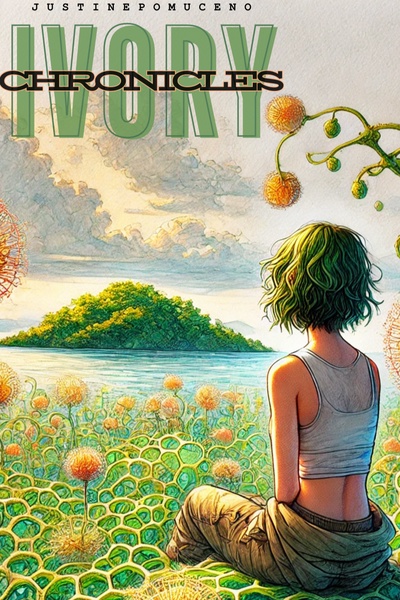This vertically aligned rectangular animated image appears to be an artistic depiction, possibly a book cover. Dominating the top of the image is the face of a young teenage girl with striking large brown eyes and slightly parted lips, revealing her top two teeth. Her shoulder-length hair has a unique grayish-green hue, and she appears to be clad in a fur coat. A backdrop of snow-covered mountains and a gray sky frames her face, enhancing the wintry setting.

Across the center of the image, an irregularly shaped tan banner prominently displays the title "Ivory Chronicles" in bold white uppercase letters. Below this central text, the scene transitions to a lower half where a tumultuous green-tinted sky looms over a crowd. The crowd comprises numerous people, some wielding weapons and others holding flags aloft, evoking an atmosphere of revolt or solidarity. The individuals at the bottom are only partially visible, indicating a mass of bodies merging into the general shading of the lower scene. The overall color palette melds tones of green, brown, red, tan, turquoise, and blue, creating a vivid and dramatic visual.